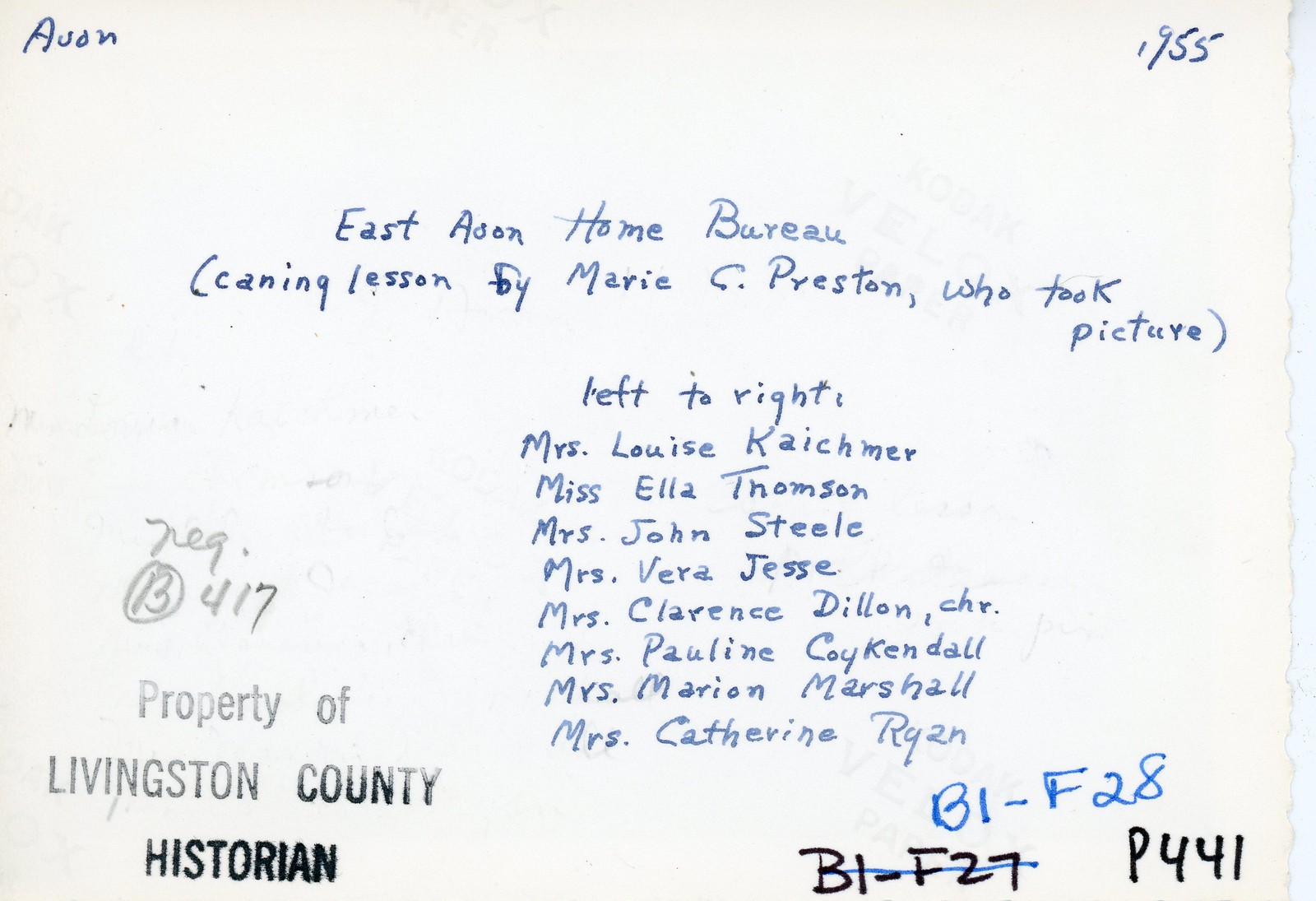This image features the handwritten reverse side of a photograph dated 1955. The note reveals the photograph documents an East Avon Home Bureau canning lesson conducted by Marie C. Preston, who also took the picture. The photograph features several individuals listed from left to right: Mrs. Louise Cashmore, Miss Ella Thompson, Mrs. John Steele, Mrs. Vera Jessie, Mrs. Clarence Dillon (identified as the chairman, denoted by CHR), Mrs. Pauline Coykendall, Mrs. Marion Marshall, and Mrs. Catherine Ryan. The writing, primarily in blue ink, also includes several reference codes and markings, such as B1-F28 and P441, suggesting updates in the cataloging system. Additionally, there is a stamp in the lower right corner stating, "Property of Livingston County Historian," indicating the photograph's ownership. Notably, the main colors in the image are black, blue, and white.